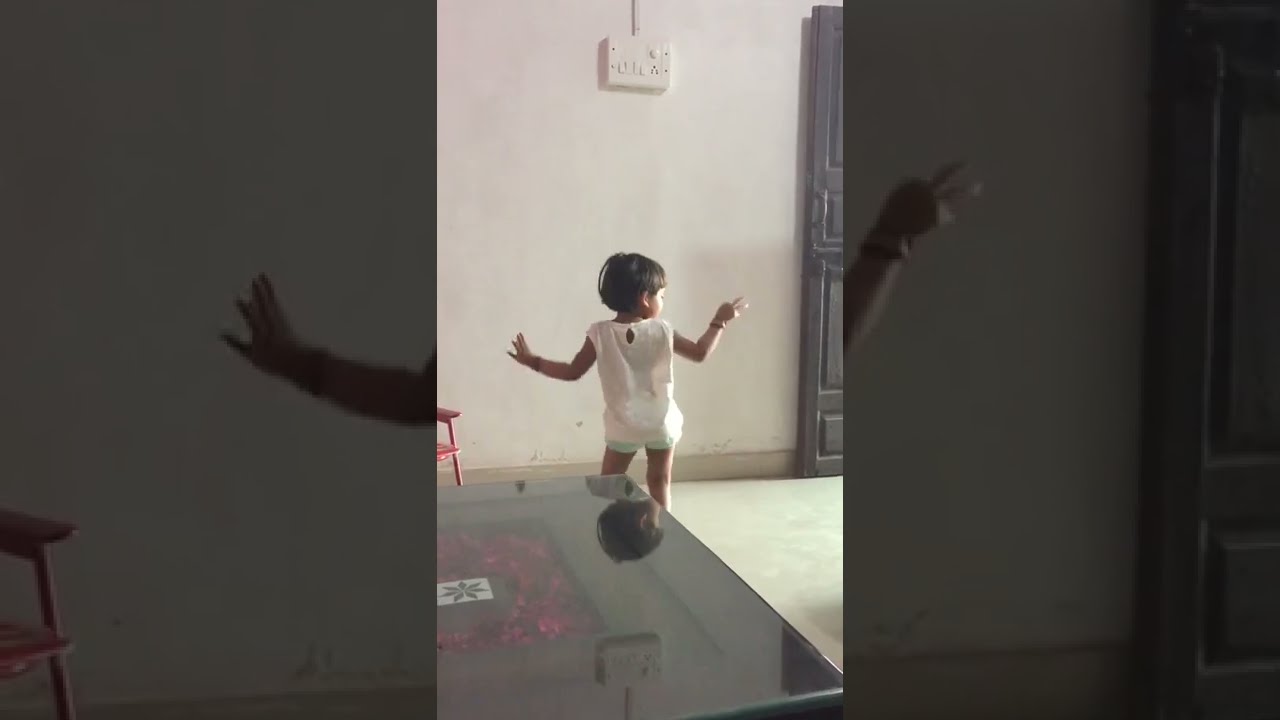In this image, we see the backside of a young child, likely between 2 to 4 years old, standing in a room. The child, who appears to be female, is wearing a loose white tank top and green shorts. She has short brown or black hair and her arms are outstretched to her sides with her head tilted slightly to the right, as if she's looking intently at something. 

Ahead of her is a glossy or glass coffee table with a shiny surface, featuring a flower design that incorporates black with magenta coloring. Adjacent to her on the left is a red foldable chair. The child is positioned against a backdrop that includes a white or beige wall with a white rectangular box, likely an electric device, mounted towards the top. The floor appears to be white, though it's unclear if it's carpet or hardwood. 

To the right of the child is a gray door, accented with etchings, that's slightly ajar with light emanating from beyond it, possibly indicating another room or an open space that's part of a house or public area. Additionally, the door on the right provides some context of the child being in a potentially public or semi-public area. Overall, the image captures a moment of curiosity and wonder as the child gazes towards the open door.